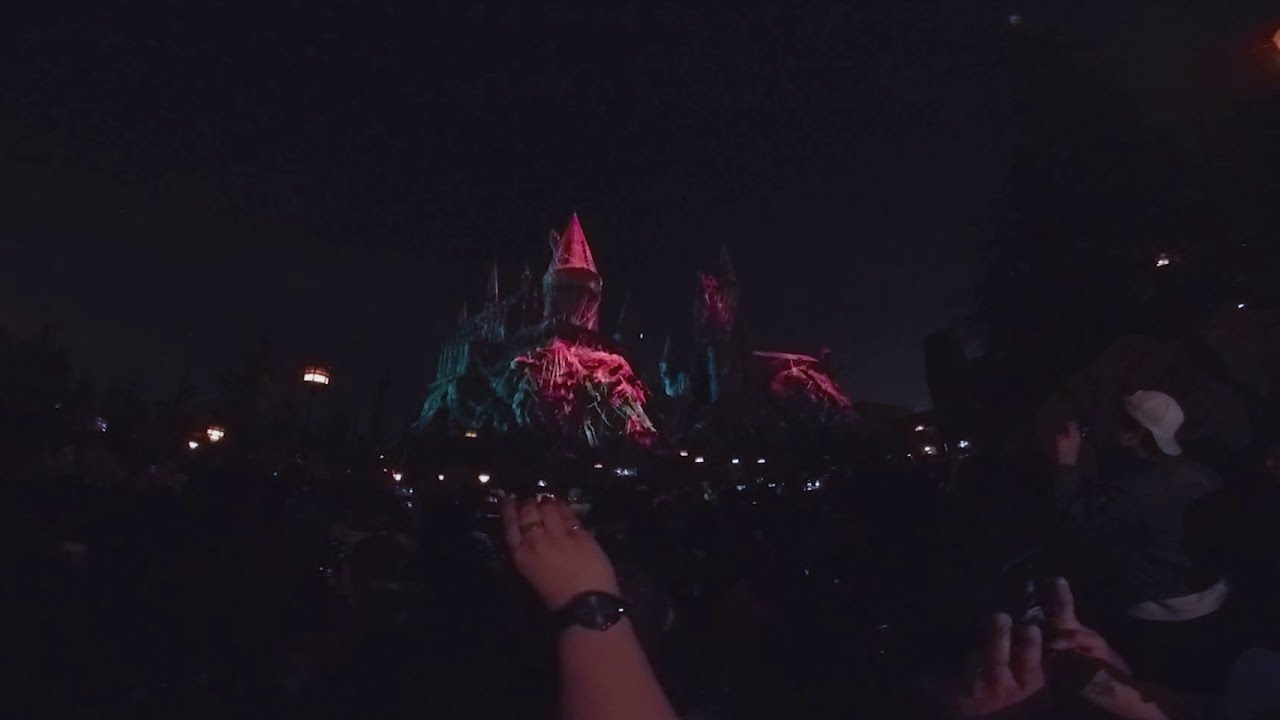The photograph captures a nighttime scene at Universal's Hogwarts Castle, which is subtly illuminated, shining in pink against a dark sky. Despite the image's poor quality and blurriness, the castle's distinctive pointy towers and rocky base are discernible. The atmosphere is lively, with a crowd gathered in anticipation, likely waiting for the renowned Harry Potter-themed fireworks and projection show on the castle facade. The scene is dotted with various soft lights from lanterns and lampposts, and numerous hands are seen extending into the frame, taking pictures with their phones. In the foreground, a Caucasian woman's arm, adorned with a watch and two rings, is visible as she snaps a photo. To the far right, a Caucasian man wearing a backward white baseball cap and sporting dark hair is also poised to take a picture, with another set of hands beside him making a similar gesture. This bustling environment, filled with eager spectators, creates an enchanting yet chaotic ambiance.